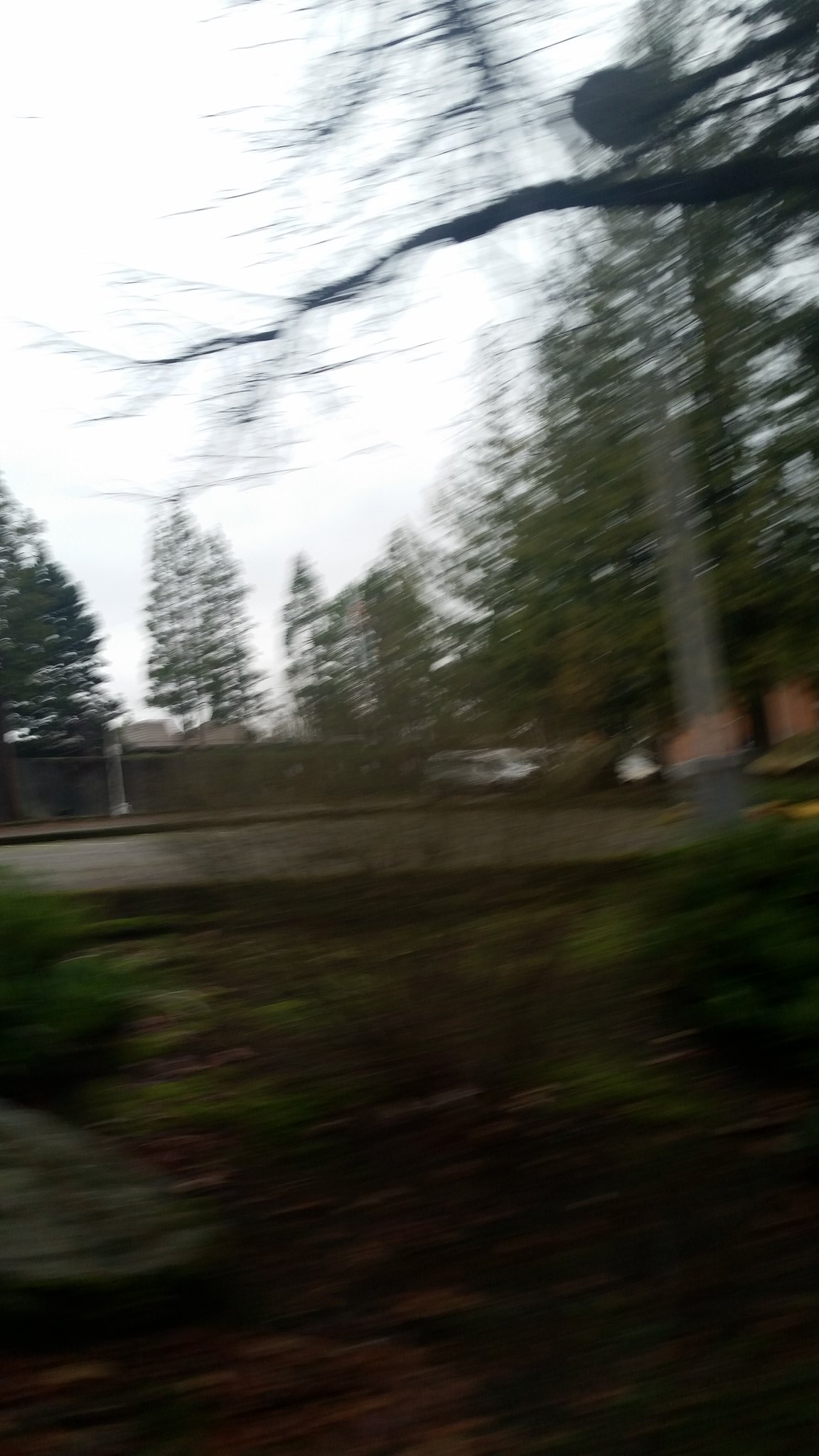The image portrays a blurry outdoor scene, most likely captured with significant motion blur, suggesting the photographer might have been moving or falling. Dominated by various shades of green and brown, the scene features a lush, vegetative area that appears almost forest-like in the foreground. In the background, tall trees with green leaves are highlighted, though there is a noticeable branch without leaves extending from the upper right corner. A sky that appears white due to the blur, possibly cloudy, forms the upper part of the image.

A large tall privacy fence is visible amongst the trees, with a white truck featuring a bed parked nearby. The scene also includes lines that give the impression of a railroad track or some sort of a bridge, adding a structural element to the view. Further examination reveals what looks like a ditch or valley area, contributing to the terrain's depth and variation. Additional details include scattered brown and green specks representing dirt, grass, and bushes. A light pole with an orange building behind it and a few indistinct, small green objects—possibly garbage cans—add to the complex blend of natural and man-made elements in this outdoor capture.